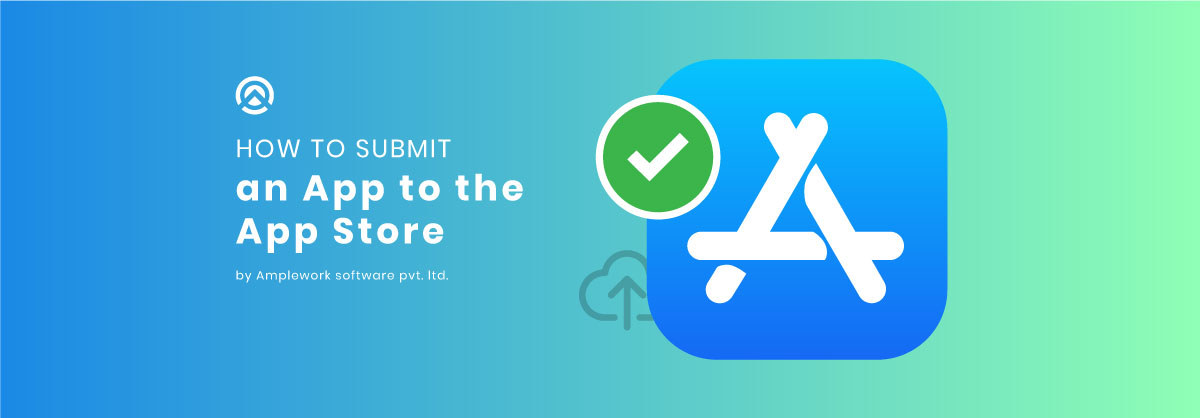This advertisement visually demonstrates the process of submitting an app to the App Store. It features a main rectangular background transitioning from blue to light blue, then to a light green, finishing with a neon green. At the center of the image is a smaller square with a blue background, bearing a minimalist icon resembling a tent made from three sticks. Adjacent to this icon is a green circle containing a white checkmark, outlined in white, denoting approval or success.

Beneath this smaller square, a black cloud-like outline with an upward-pointing arrow runs through the middle, indicating uploading or submission. On the left side of the image, written in white text, is the title “How to Submit an App to the App Store” by Ampleworks Software Pvt. Ltd. Above this text, there is a unique emblem comprised of concentric circles — a blue circle within a white circle, and a pyramid-like design originating from the left and right, converging at the bottom center of these circles.